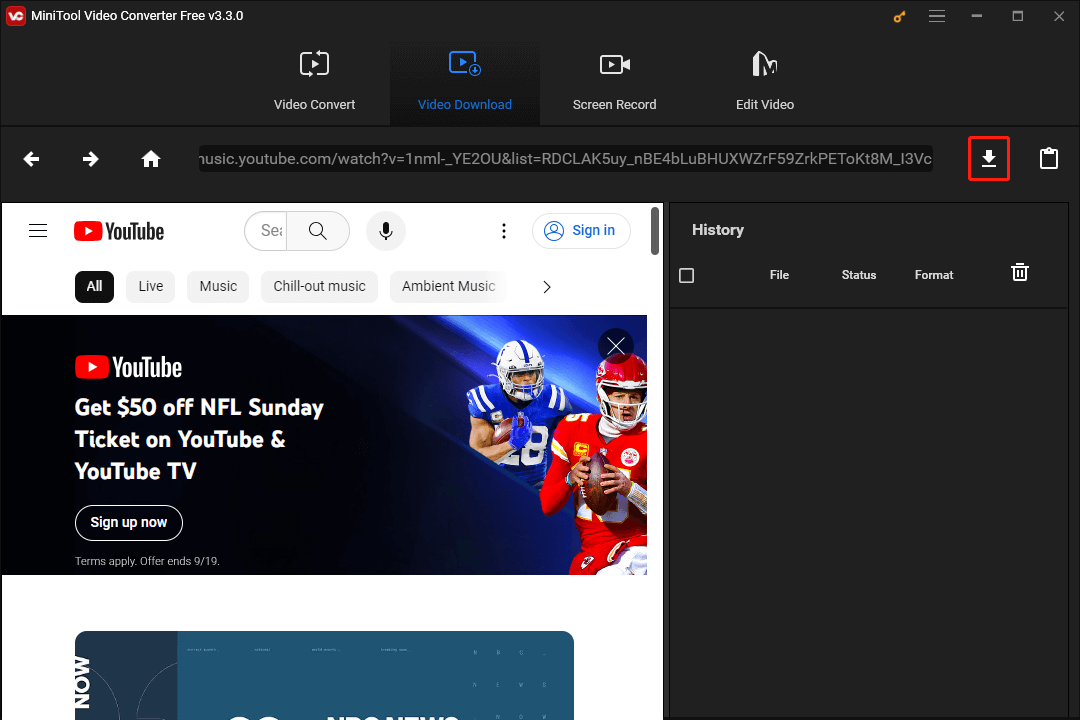Screenshot Description: 

The screenshot portrays the user interface of MiniTool Video Converter Free v3.3.0, featuring a dark gray background that dominates the visual theme. At the top left corner, the software name is prominently displayed alongside a square red logo bearing the initials "VC". Adjacent to this title, on the right side, a series of icons are arranged: a yellow key icon, a three-bars menu icon, followed by the standard window controls for minimize, maximize, and close.

Beneath this top bar resides a row of four multifunctional buttons, each with both an icon and corresponding text: "Video Convert," "Video Download," "Screen Record," and "Edit Video." This layout provides easy access to the main features of the software.

Adding to the interface's accessibility, an element resembling a browser bar is present. It includes navigation buttons for "Back," "Forward," and "Home," accompanied by a URL input field. Directly to the right of this bar, a red-outlined "Download" button stands out, alongside a clipboard icon.

The lower section of the screenshot displays a YouTube page, visible in the bottom left quadrant, indicating that the software might be interacting with the content or downloading from the platform. The cohesive layout and intuitive iconography ensure streamlined usability for the user.